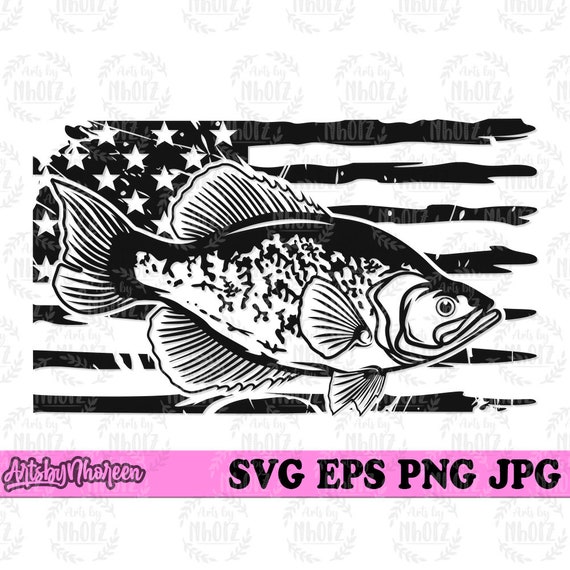This is a detailed black-and-white sketch overlay of an American flag and a fish, framed in a painterly style. The flag features black stripes on a white background with a black canton and white stars. A bass swims from left to right, positioned centrally over the flag's stripes and stars. The fish is depicted in a side view with black and white speckles, a fin on its back and belly, and its mouth slightly open, showing a single visible, black-colored eye. In the bottom left corner, a cursive script that seems to say "Arts by Nahreen" is difficult to read. Below the image, a purple banner stretches from left to right, with bold black text listing photo designations: SVG, EPS, PNG, and JPG. The artwork includes illegible watermarking stamps.